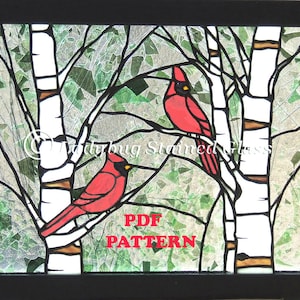The image appears to be a detailed PDF pattern for a stained glass template, featuring a vibrant outdoor scene with two striking cardinals. The scene is framed by horizontal black bars at the top and bottom, with the top bar slightly uneven, thinner on the left and wider on the right. The cardinals are perched on the white and brown trunks of what seem to be aspen or birch trees. The cardinal on the left, with a yellow beak, sits on a branch diagonally oriented so its head points toward the upper right corner, while its tail points toward the bottom left corner. The right cardinal, with a gray beak, perches on a forked Y-shaped branch, looking down towards the bottom right corner. Both birds display rich red feathers, with the cardinal on the right featuring a touch of black around its face. Surrounding the birds are branches with leaves in varying shades of green and gray, set against a green and cream background. A watermark at the bottom in red reads "PDF pattern," with additional text possibly indicating "Fitchburg Stained Glass."